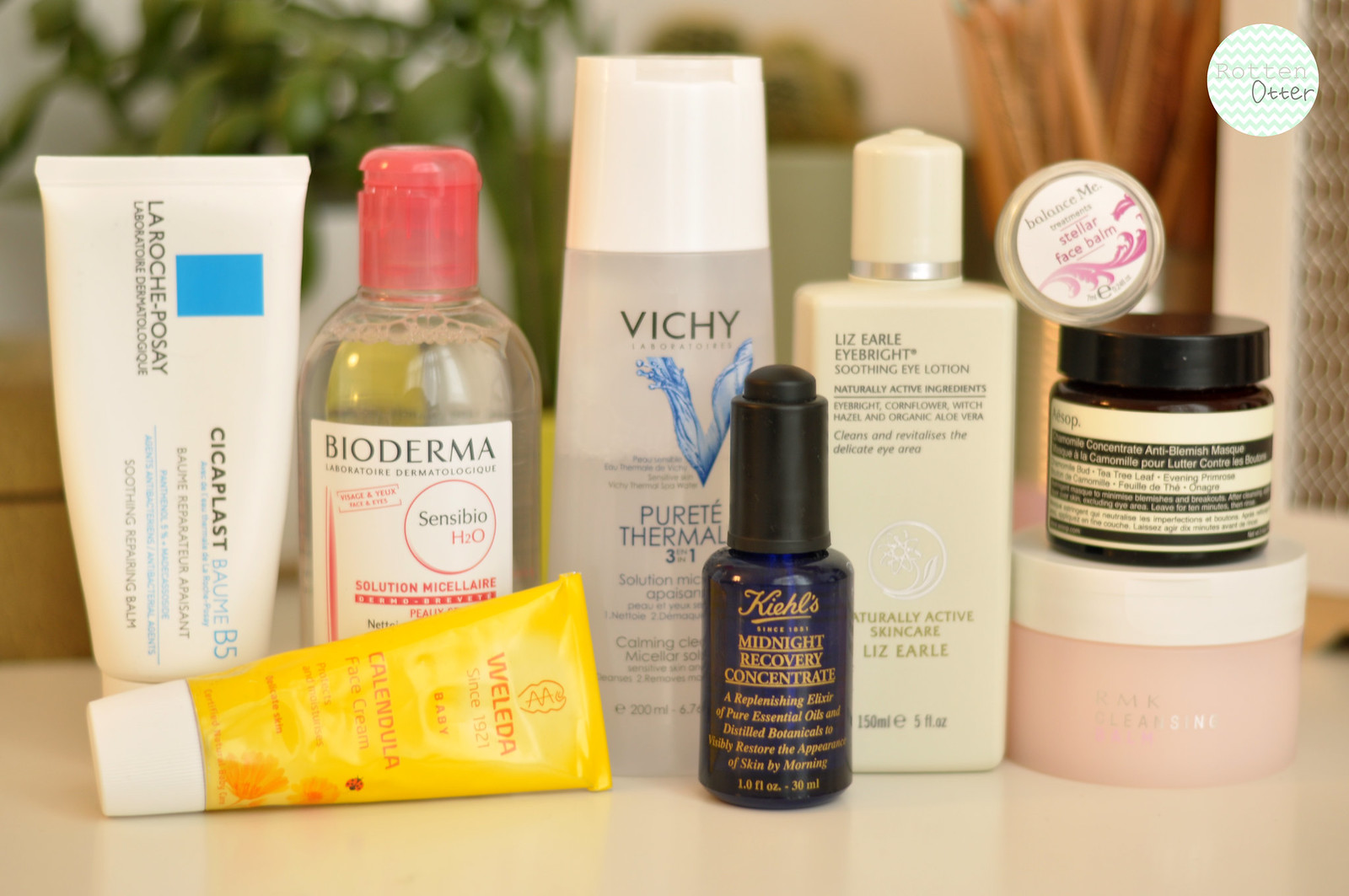On a spa-like counter adorned with bamboo furniture and lush greenery sits an exquisite collection of skincare products. The serene atmosphere is captured in the photo, which features a slightly blurred background, enhancing the focus on the products. In the top right corner of the image, there's a circular logo with the words "Rotten Otter" against a white and green chevron patterned background.

From left to right, starting at the back, the first product is a white squeezy container labeled La Roche-Posay Cicaplast Baume B5, a soothing and repairing balm. Next to it is a clear, round plastic bottle with a white label and a pink flip cap, identified as Bioderma Sensibio H2O, a micellar cleansing water.

Beside it, there is a clear and white plastic squeezy bottle from Vichy, named Pureté Thermale 3-in-1, another calming micellar solution. Following that is a rectangular, yellow-tinted hard plastic bottle with a round cap, labeled Liz Earle Eye Bright Soothing Eye Lotion, featuring naturally active ingredients like eyebright, cornflower, witch hazel, and organic aloe vera.

Adjacent to this is a small circular container with the label Balance Me Stellar Face Balm. Below it sits another round container, black with white text, from Aesop, marked Chamomile Concentrate Anti-Blemish Mask, containing chamomile bud, tea tree leaf, and evening primrose.

The shelf also includes a pink and white round container, slightly out of focus, known as RMK Cleansing Balm.

In the front row, starting from the left and laying on its side, is a yellow squeezy container of Waleida Calendula Face Cream, designed for delicate skin, and lastly, a small dark blue round bottle with a black cap, likely a dropper, identified as Kiehl's Midnight Recovery Concentrate, an elixir of essential oils and botanicals aimed at visibly restoring skin by morning.